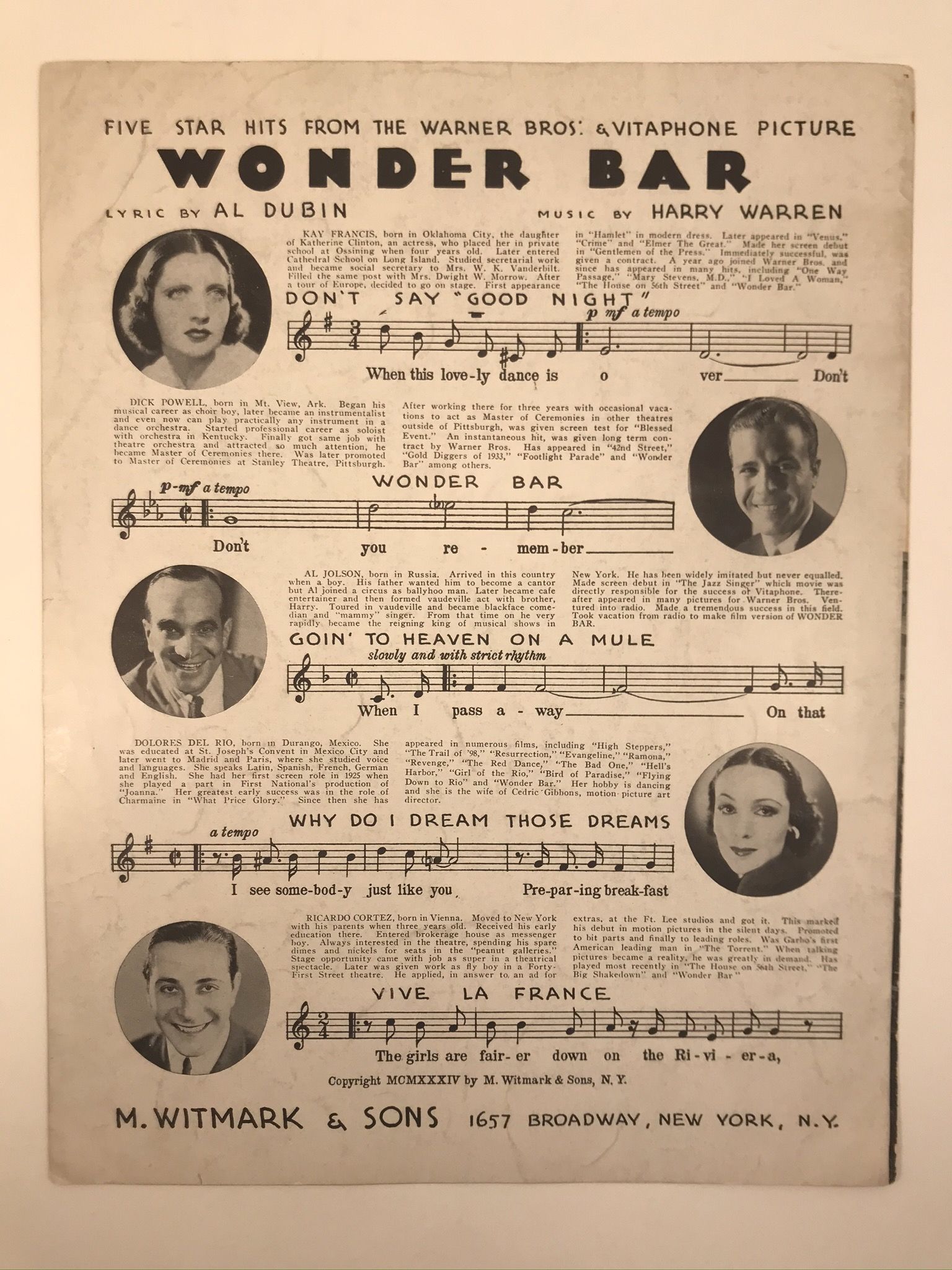This image showcases a vintage magazine or newspaper ad, possibly the back of a Broadway program, featuring "Five Star Hits from the Warner Brothers and Vitaphone Picture, Wonder Bar." The piece is likely in black and white, although one description mentions a faded pink hue, and is filled with extensive, small text detailing the content. Dominating the top of the ad is the bold title "Wonder Bar," with credits to lyricist Al Dubbin and composer Harry Warren. The page displays five circular portraits of composers or performers, each accompanied by music notes, song titles, and brief descriptions. At the bottom, the address "M. Whitmark and Sons, 1657 Broadway, New York, New York" is prominently displayed, confirming its connection to a prominent New York music publisher. The overall aesthetic suggests an early 20th-century setting, capturing a rich piece of musical and theatrical history.